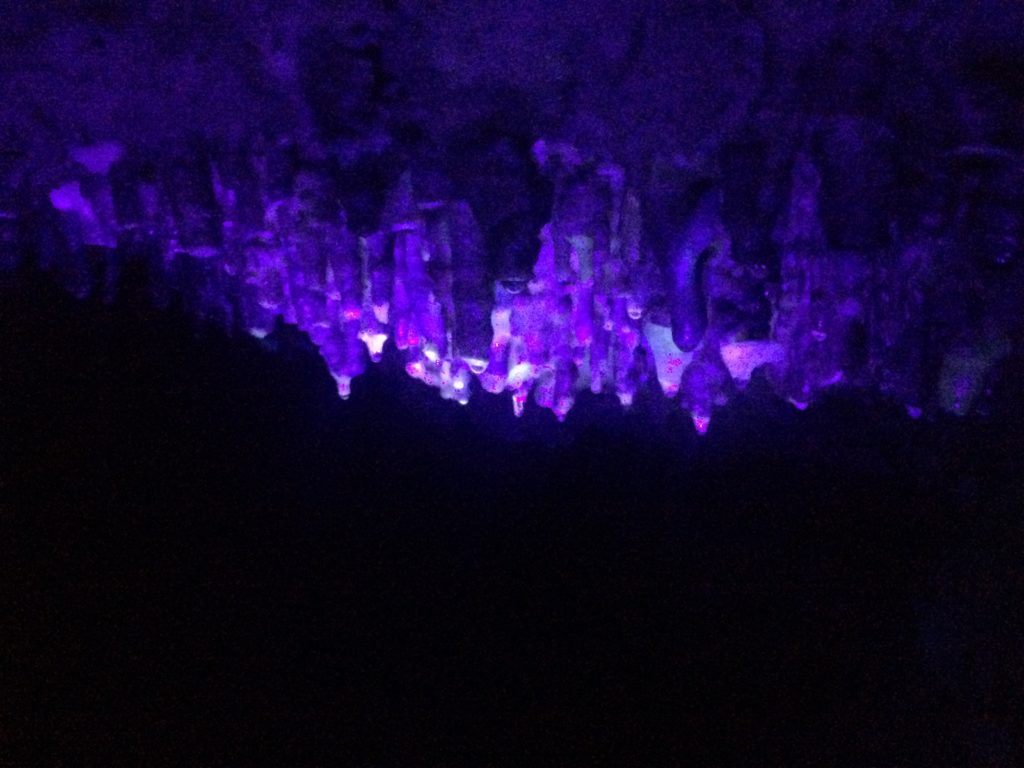The image depicts a dark cave interior illuminated by a striking purple glow emanating from an array of crystal formations hanging from the ceiling. The crystals, which have a pointed, almost cylindrical shape reminiscent of stalactites, are primarily concentrated in the top half of the picture, with their tips extending into the empty black space below. This black void comprises the entire bottom half of the image, highlighting the sharp contrast between the glowing crystals and their surroundings. A range of colors can be seen in the crystals, transitioning from a bright whitish purple at the center to darker purple hues towards the edges. Some of the crystals are partly obscured by dark, rocky outcroppings, adding to the mystique of the scene. The uneven arrangement of the crystals and rocks, where the left side appears closer to the cave's ceiling and the right side extends further downward, enhances the organic and rugged appearance of this subterranean landscape.